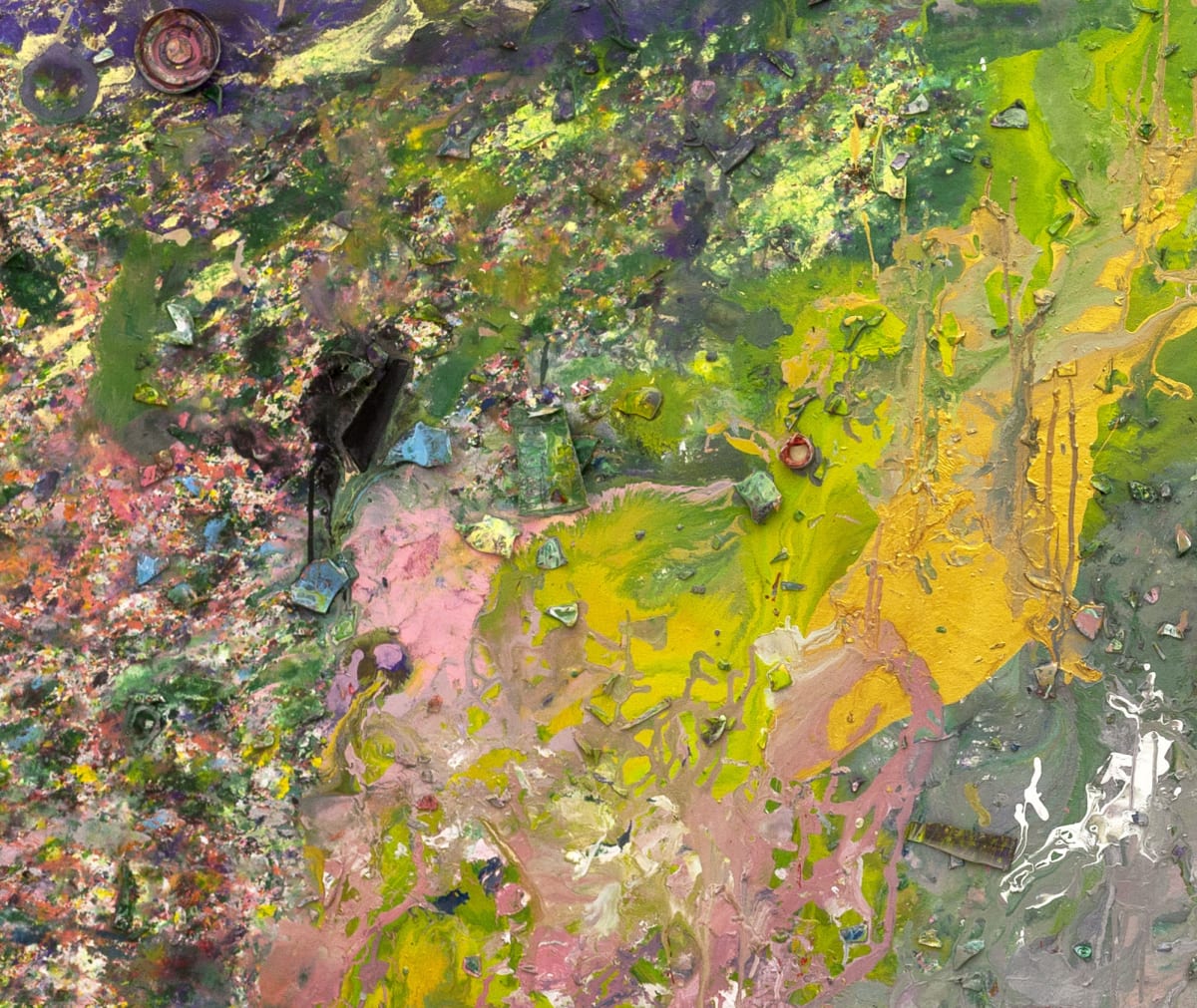This image depicts an abstract work of art often referred to as splash or spray art, where paint is dynamically splattered and sprayed onto the canvas. The artwork is a busy, multi-colored composition featuring a spectrum of hues including turquoise, blue, pink, yellow, green, red, white, and purple, creating a visually chaotic yet vibrant appearance. Notably, the canvas includes various textures and materials, such as particles of what appears to be broken glass and pieces of clay or pottery, which have been attached to the surface, adding depth and complexity to the piece.

In the lower right corner, substantial areas of solid colors are present, predominantly featuring a blend of grayish-green, yellow, yellow-orange, and yellow-green tones which then transition into deeper greens and blue-greens as one moves across the canvas. The top right section is characterized by smaller splatters and droplets, giving a messier and more intricate feel to that part of the composition.

The left side of the image is dominated by a multitude of mixed colors and debris, evoking a sense of looking down at a chaotic trash yard or dump site, with colors and materials seemingly scattered at random, enhancing the abstract nature of the piece. The overall effect is one of dynamic energy and complexity, with no discernible text or writing present anywhere in the artwork.